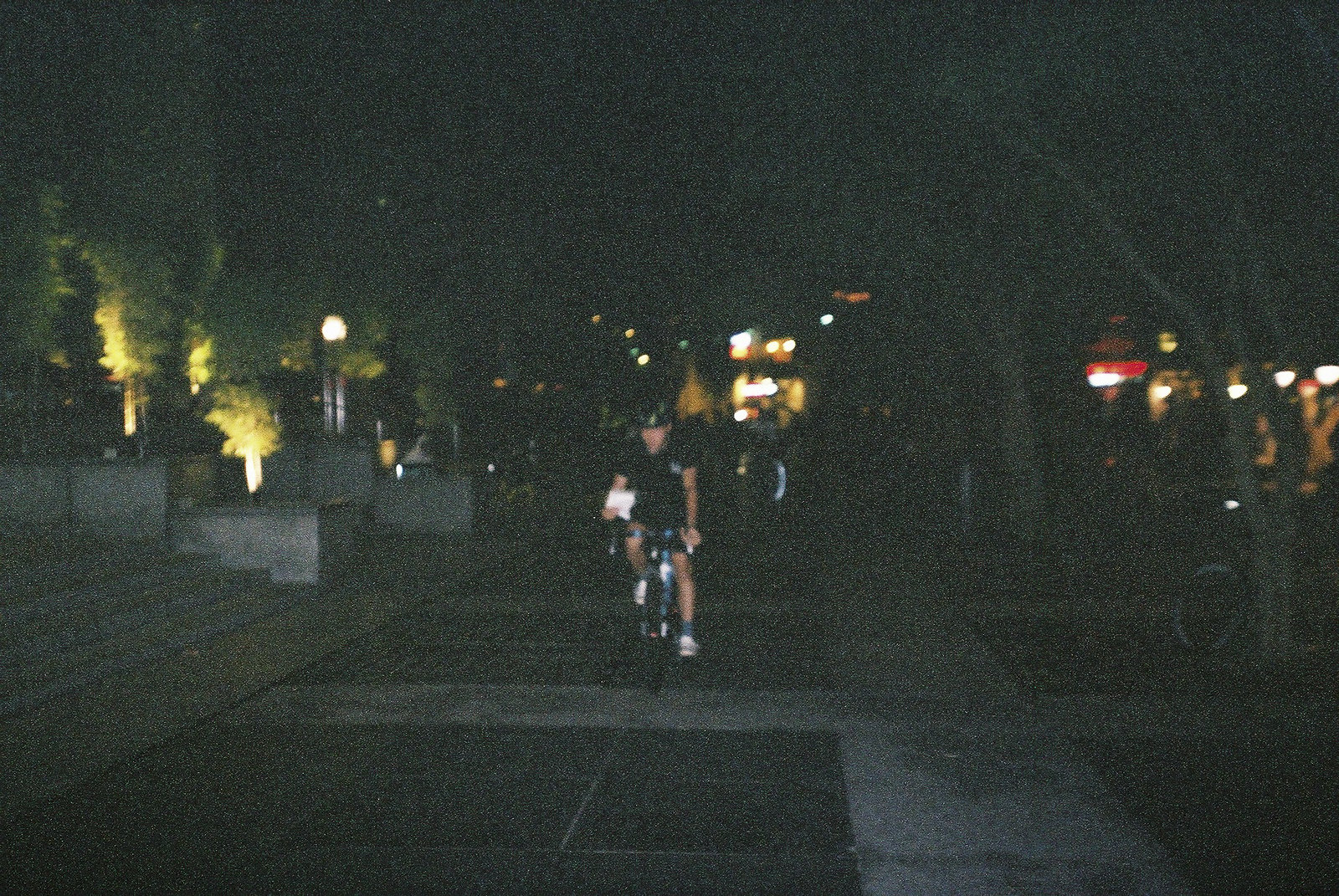In this dimly-lit nighttime photograph, a person is seen riding a bike on an exceptionally wide sidewalk that hints at it being part of a college campus or a similar large public area. The cyclist, moving towards the viewer, is predominantly silhouetted against the sparse light. On the left side of the image, cement steps ascend towards an unknown structure, illuminated by a couple of faint lights. Across the street to the right, lights from what appears to be businesses are visible, alongside the dark outlines of trees lining the street. In the distant background, additional lights dot the end of the wide sidewalk. The cyclist appears to be holding something white in their right hand, although its details are obscured due to the lack of flash.